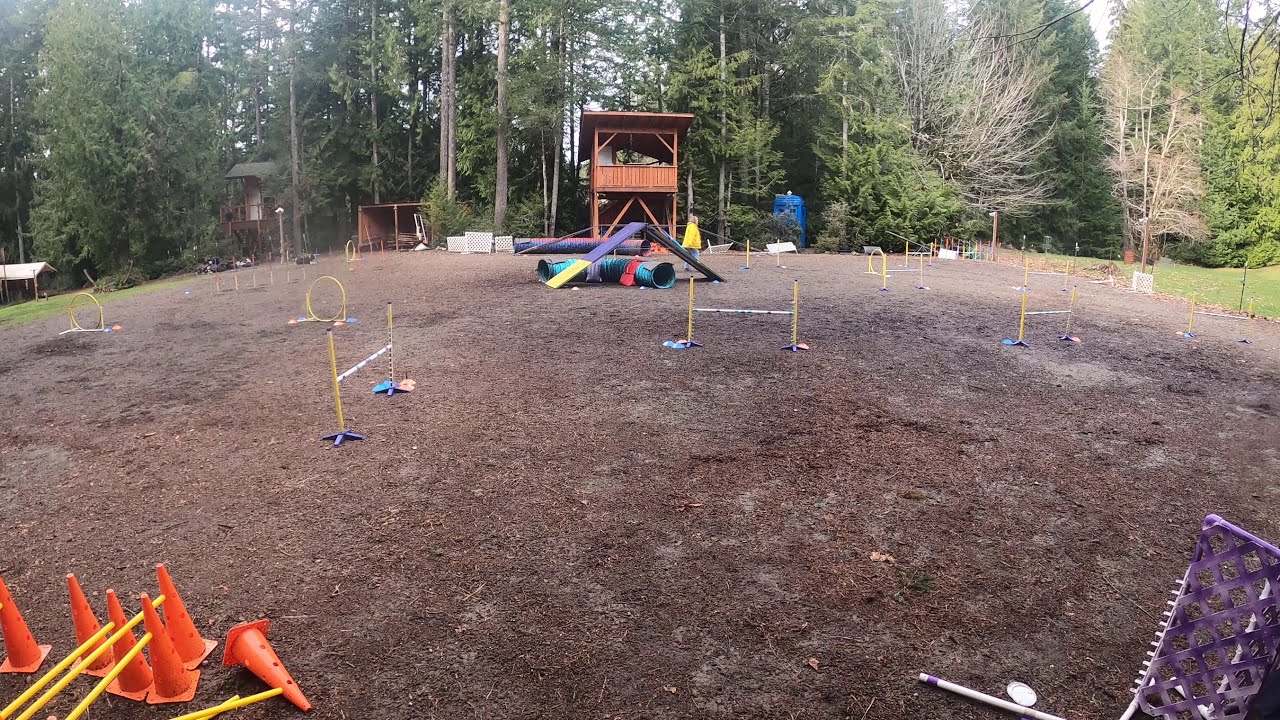This image depicts a flat, expansive dirt field covered with patches of dead grass. Along the left corner of the field stand six orange cones with four yellow sticks extending through them. On the right side, a cart or net with purple netting and white frames can be seen. The field is also dotted with yellow skinny poles connected by white lines, along with yellow hoops lying on the ground. A tent cover in vibrant colors—purple, yellow, and turquoise—adds a splash of brightness, accompanied by a tube in matching hues.

In the center, a wooden lookout structure with a small roof rises above the field, suggesting a place for spectators or judges. The background is dominated by a dense line of tall trees, providing a natural border to the field. Towards the back, there is some sparse greenery. This setup, complete with various bars, ramps, and hoops, strongly resembles an obstacle course typically used for dog competitions or training, supported by the assortment of agility equipment spread across the area.